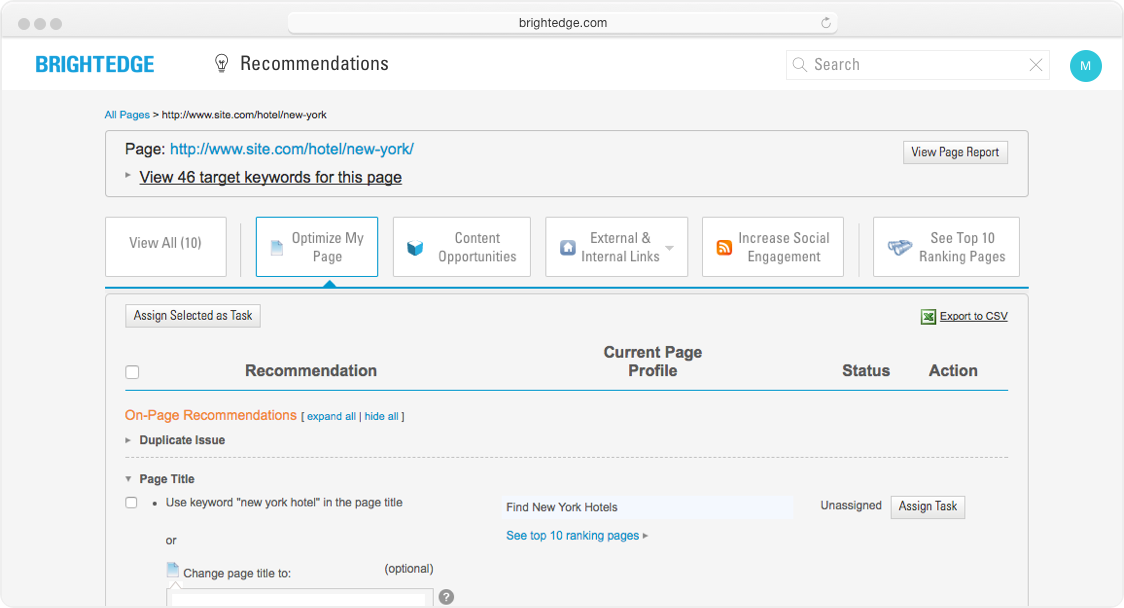Here is a detailed and cleaned-up version of the caption:

---

The image features a user interface with a gray background and various highlighted elements. At the top, there's a bright blue edge displaying the word "Recommendations" in black. Underneath that, a search bar is visible, accompanied by a blue circle containing a white "M."

The interface prominently displays two main divisions: "All Pages" and "Website," both labeled in blue. Below these divisions, there's a gray rectangle that includes the text "View Page Report" in black. The section also offers the option to "View 46 Target Keywords for This Page" and "View All Keywords," each highlighted with a blue triangle arrow directing towards the "Optimize My Page" option.

Additional features include sections for "Content Opportunities," "External and Internal Links," and tools to "Increase Social Engagement." There's also an option to "See Top 10 Ranking Pages."

Towards the bottom, command buttons are presented in gray rectangles, such as "Assign Selected as Task" and "Export to CSV." 

The recommendations area comprises several columns labeled "Recommendation," "Current Page Profile," "Status," and "Action," with on-page suggestions highlighted in orange. Blue-text options for "Expand All" and "Cut All" are also included.

A specific recommendation highlights a duplicate issue. It suggests using the keyword "New York Hotel" in quotation marks within the page title.

---

This caption provides a comprehensive and coherent description of the image, detailing its various sections, colors, and functionalities.